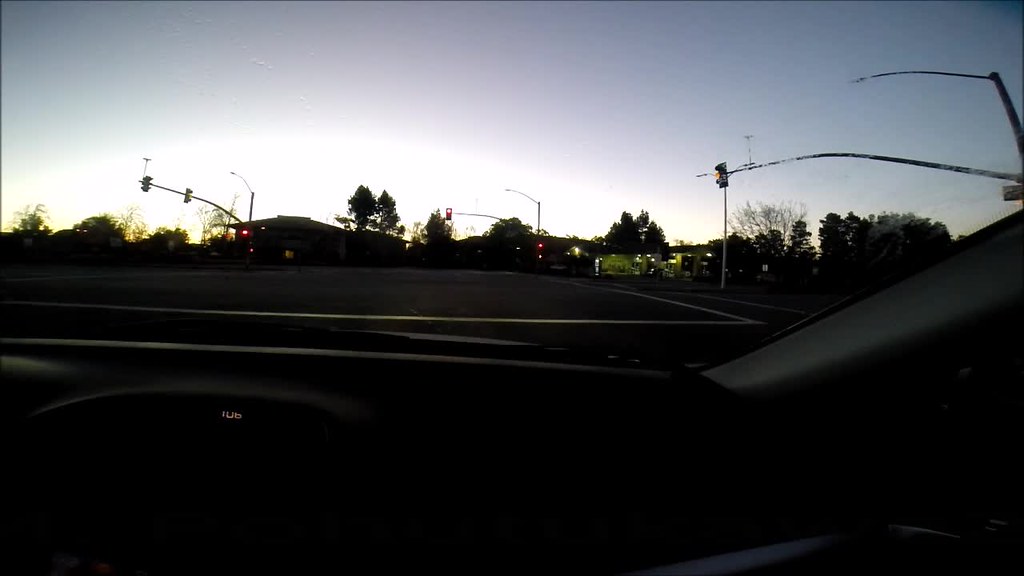This color photograph, likely taken around dawn or dusk, offers a serene view from the interior of a car, presumably through the driver's side window. The scene unfolds within an empty parking lot, devoid of any vehicles. At the far edge of the parking lot, dim lighting creates near-silhouettes of houses and numerous trees, adding a touch of tranquility to the image. The sky above transitions from a deep gray at the top to a lighter hue near the buildings, suggesting the onset or end of daylight. The setting appears to be near an intersection, with pairs of traffic lights visible on both the left and right sides of the frame, and an additional traffic light situated on the far right.